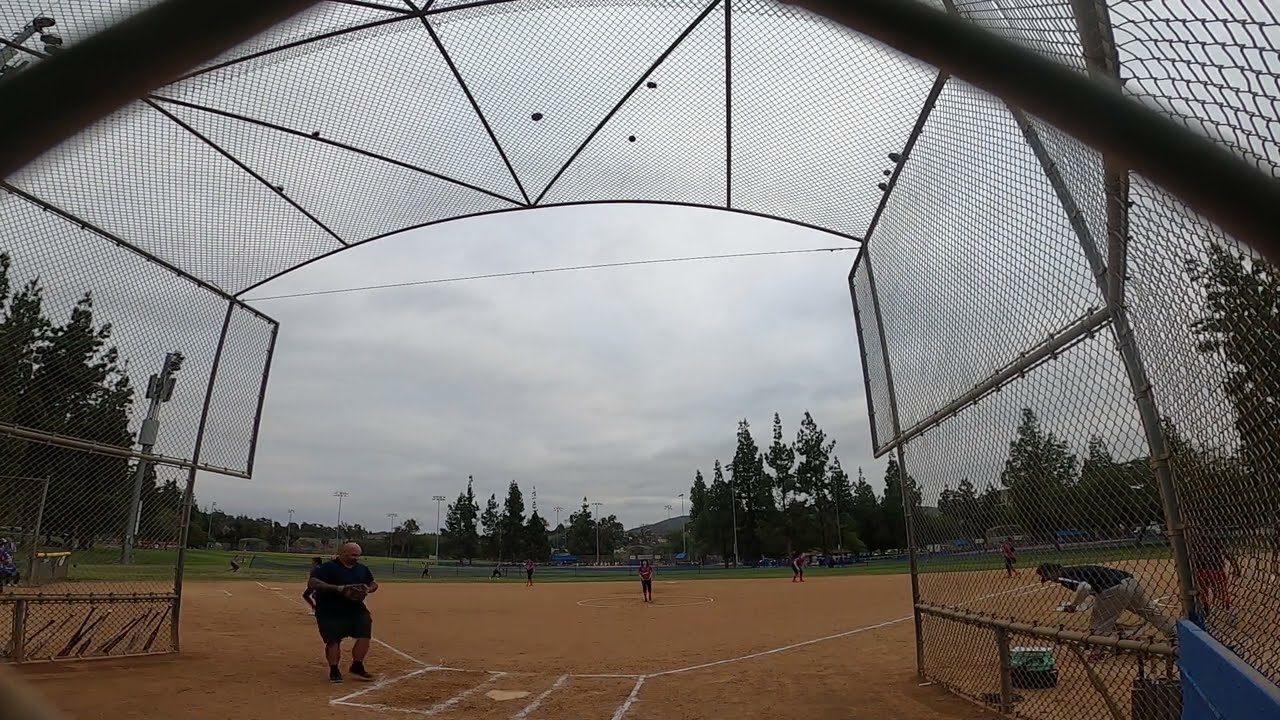The photograph is a detailed color image captured from the point of view of someone behind a chain-link fence, likely taken inside a warm-up area or dugout looking onto a small baseball field. The scene centers on a typical brown sand baseball diamond marked with white painted lines indicating the bases and other important spots. The overcast gray sky looms above, casting a muted light on the field. You can spot several players on the field, including a central figure on the pitcher's mound and a few others scattered around. To the right side, a man, dressed in a dark t-shirt and long dark trousers, is seen picking up items from the ground, possibly equipment. On the left side of the image, a row of baseball bats leans against the chain-link fence. There is also an older man near the diamond, wearing a t-shirt and shorts, facing sideways, and possibly offering instructions or observing the play. In the distance beyond the outfield, a line of trees is visible along with additional fencing, perhaps indicating the boundary of the field. The atmosphere suggests an active game or practice session, capturing the essence of a community baseball or softball game on an overcast day.